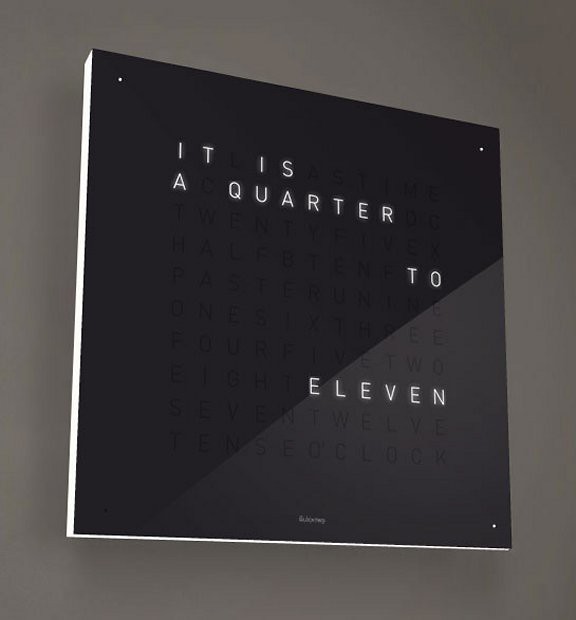This photograph features a framed picture mounted on a gray wall. The picture itself has a predominantly black background with a white capitalized font that reads: "IT IS" on the first line, closely followed by "A QUARTER" on the second line. The phrase "A QUARTER" has slightly more spacing below it, leading to the word "TWO," which is aligned to the right. Significantly spaced beneath "TWO" is the word "ELEVEN," also right-aligned. In the bottom center of the picture, there's a small, indecipherable white text. Notably, three of the picture's corners—top left, top right, and lower right—feature white dots, while the lower left corner does not. The picture appears to be set within a matted frame, with the white mat noticeably visible along the left and bottom edges.